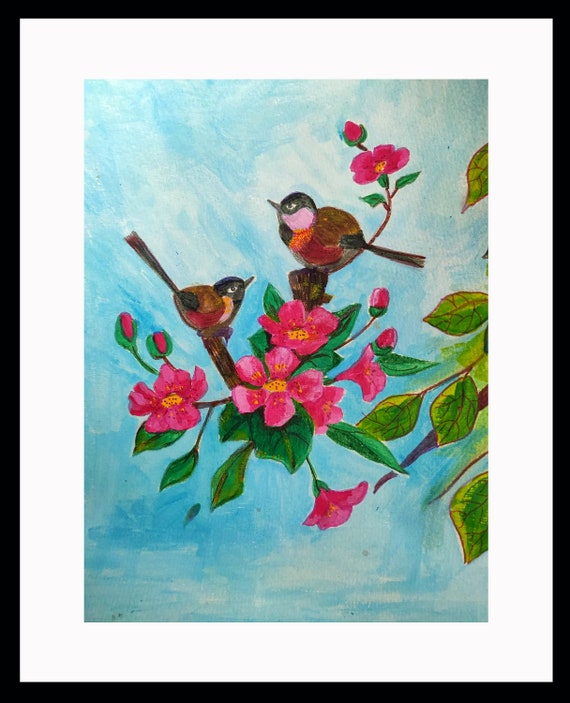This is an image of a highly detailed and stylized painting, possibly created with colored pencils, depicting two birds perched on floating branches adorned with blossoms. The painting is set against a blue backdrop, which transitions from darker blues and grays at the bottom to lighter blues and whites at the top, suggesting a sky. It is encased in a black frame with a white inner border, accentuating its delicate details. 

The two birds in the painting have intricate coloring: they both feature black heads, with the bird on the left displaying lavender cheeks and a dark brown tail with a white tip, while the bird on the right has orange accents on its cheeks and a black tail. Both birds sport brown bodies with varying underbelly colors; the left bird has a red underbelly, and the right one has a black underbelly. Pink, green, and yellow hues dominate the blossoms and leaves on the branches, which enhance the ethereal feel of the artwork as they appear to float in mid-air, unconnected to any visible tree trunk.